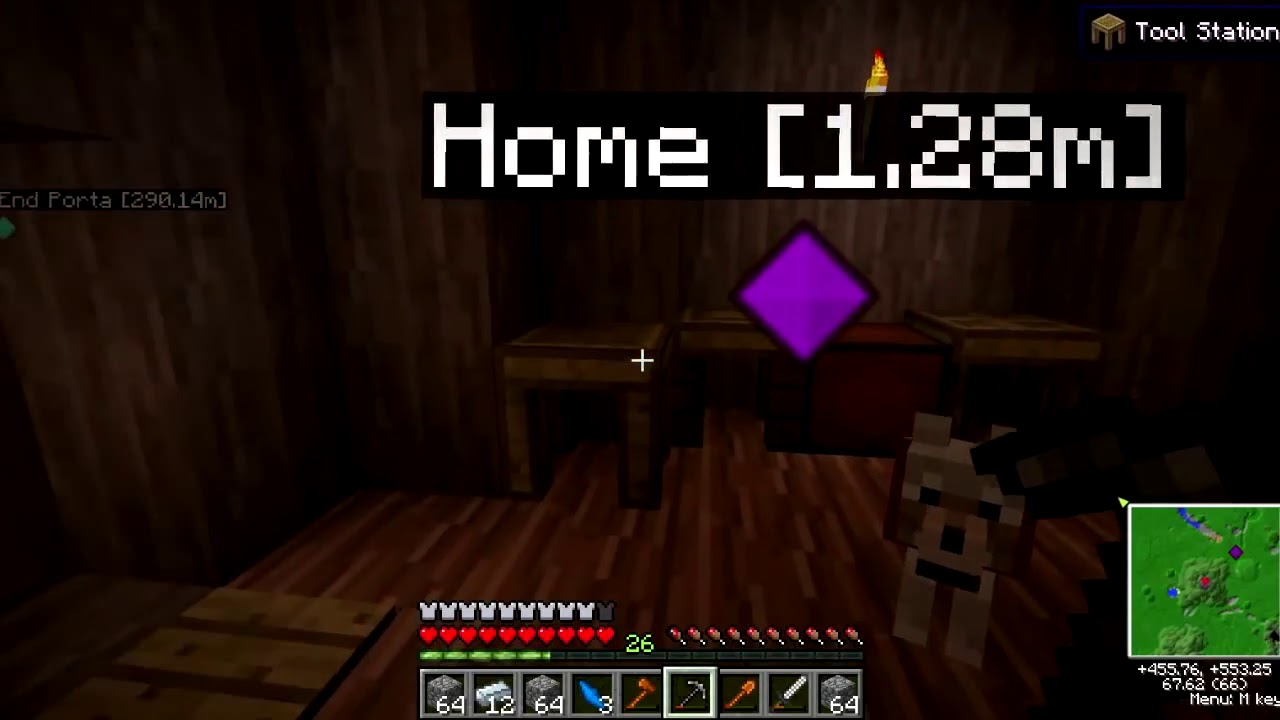This is a detailed screenshot from the video game Minecraft, showcasing a player’s in-game environment within a wooden cabin-like room. The scene features tables against a wall with a small brown, bear-like or dog-like figure situated in the lower right-hand corner—possibly the player's companion. Dominating the center of the image, there is a purple diamond underneath a waypoint indicator that reads "HOME (1.28m)" in prominent white letters. Close to the top-right, there's a black rectangular block labeled "Tool Station" next to a small brown stool.

The user interface is filled with significant details: On the left, a black background with the text “END PORTA (290.14m)” is visible. The bottom-right corner contains a green topographical map with various coordinates inscribed beneath it, and labeled “MENU: M KEY.” Centrally located at the bottom of the screen is the player’s HUD, displaying a health meter with red hearts for lives, a white T-shirt-like health status bar, and a progression meter. Below these, the player's inventory is shown, featuring nine square boxes for power-ups, the current score of 26, and a green progress bar partially filled. This vivid depiction encapsulates the Minecraft aesthetic and showcases the detailed elements of the game's interface and environment.